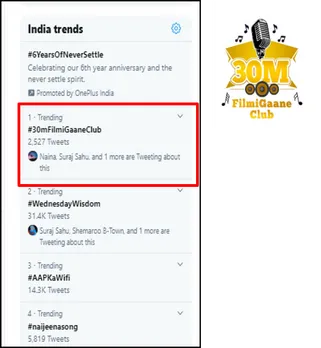The image showcases a small screen at the top featuring the "India Trends" section. At the top of the screen, a prominent headline reads: "Six Years of Never Settle: Celebrating Our Six-Year Anniversary at the Never Settle Spirit." Below this, a notification indicates the content is "Promoted by OnePlus India." 

Highlighted with a red box, the "Trending" section reveals:
1. "Filmy Gain Club" with 2,527 tweets; multiple users like Nina, Siraj, Sahoo, and others are engaging in discussions under this topic.
2. "Wednesday Wisdom" is listed as the second trending topic, garnering 31.4K tweets.
3. A cryptic string "APKAW," with "APK" and "W" in capital letters and "a" in lowercase, has 14K tweets.
4. The fourth trending spot is occupied by the hashtag "NAIGE," with 5,819 tweets.

The background transitions subtly between very light gray and white, making it challenging to distinguish the exact boundaries. On the top right corner, a golden microphone icon is visible, indicating 30 minutes, and "Filmy Gain Club" is highlighted in gold at the bottom.